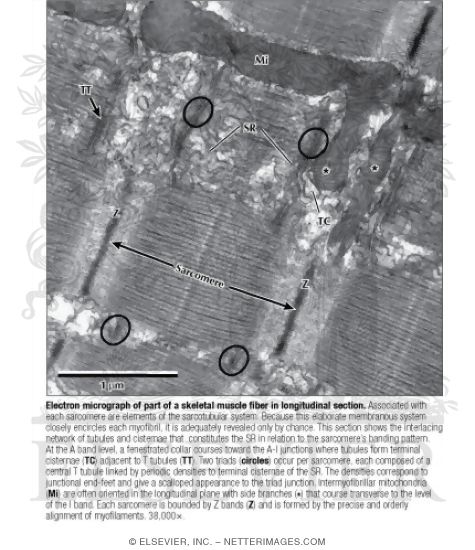This black-and-white electron micrograph presents a detailed longitudinal section of a skeletal muscle fiber. The image prominently features labeled components, including the sarcomere, a crucial structural unit of muscle fibers. Several arrows point to specific parts of the muscle fiber, notably labeled as TT, MI, SR, TC, and Z. These labels highlight elements of the sarcotubular system, which closely encircles each myofiber. The muscle fiber segmented areas contain distinct white patches marked with these abbreviations, aligning with various parts of the muscle structure. In each corner of the diagram, there are black circles with letters, set against a gray and white background. Below the image, a caption in small black letters reads: "Electron micrograph of part of a skeletal muscle fiber in longitudinal section," followed by an explanation detailing the sarcotubular system's relevance and the intricate labeling showcased.